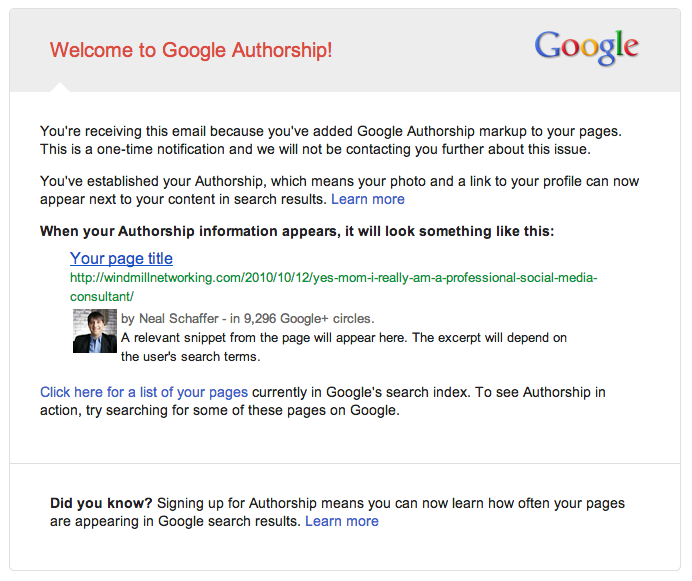The image depicts a screenshot of a Google Authorship notification email. At the top left corner, the email headline reads "Welcome to Google Authorship." On the right side, there's a Google logo. The main body of the email informs the recipient that they received this notification because they have added Google Authorship markup to their web pages. It mentions that this is a one-time notification and that no further contact will be made regarding this matter.

The email explains that by establishing authorship, the recipient's photo and a link to their profile can appear next to their content in search results, providing a visual example of what this looks like. The example includes a mockup showing a page title, its URL, a photo of a gentleman in a suit with a blue button-down shirt (no tie), the author's name, and the number of Google+ circles they are in. A relevant snippet from the page is also shown, stating that the excerpt displayed will depend on the user's search terms.

The recipient is encouraged to click a link to see a list of their pages currently indexed by Google and to try searching for some of these pages to see the authorship in action. The tone and layout of the email indicate that it's an official communication from Google to guide the user through the benefits and visual impact of Google Authorship.